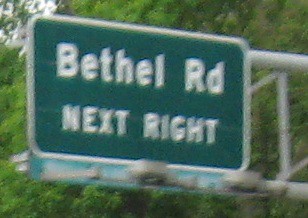This photo captures a somewhat grainy but discernible street sign positioned high in the air on a horizontal, rounded white pole. The green and white sign reads "Bethel Rd" with "Rd" being the abbreviation for "Road." Below this, an additional smaller sign indicates "Next Right." Daylight illuminates the image, revealing spotlights beneath the sign, suggesting they are used to illuminate the sign at night. The background is dominated by a lush expanse of tall, verdant trees, towering above the sign and adding a touch of nature to the urban setting.